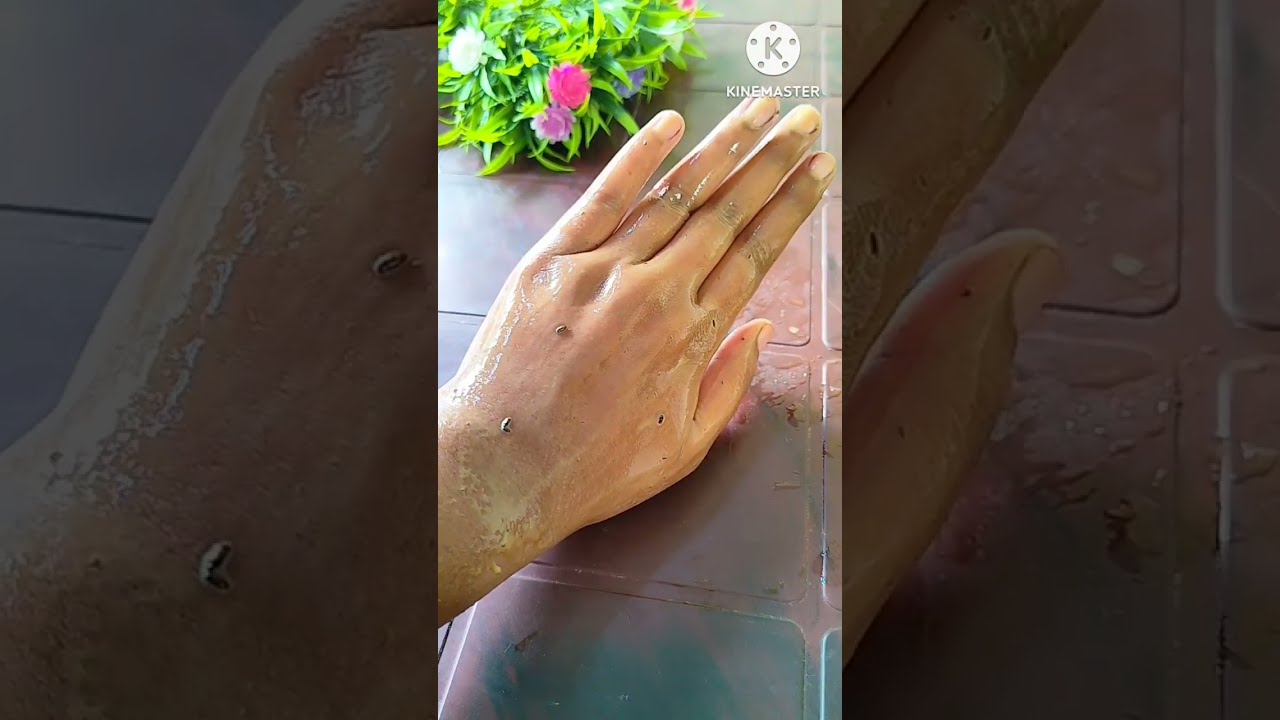The image is a vertical photo likely taken from a phone, featuring a slender, possibly female left hand. The hand, which has a light brown tone and is covered in an oily liquid, appears glossy. It's positioned with all five fingers facing upward towards the top right corner. The surface beneath the hand consists of dark brown and dark pink tiles. There are a few specks on the hand that resemble insects or black bumps, almost like ticks or scars, with the close-up sections on the left and right highlighting these details—the left showing the side of the hand and the right focusing on the thumb. Above the hand, in the upper left corner, there's a plant with green leaves, a pink flower, a purple flower, and a white flower. In the top right corner, a logo displays a white circle with the letter "K" at its center, surrounded by five dots, and the text "K-I-N-E-M-A-S-T-E-R" beneath it.